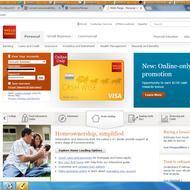Screenshot of a vintage website on a Windows desktop, showcasing a low-resolution, pixelated image that highlights an outdated web design. The primary color scheme is blue, orange, and white. At the top of the screenshot, multiple tabs are visible—seven in the first row and five in a secondary tab layer, demonstrating an unusual double-layer tab setup.

In the center of the page, there is an image of a Visa card, notable for its yellow color and a red square in the top-right corner. To the right of this, a blue box contains the text "New Online Only Promotion." Adjacent to the Visa card on the left is an orange box with fields that appear to be for user login.

Below the Visa card, a lengthy text block is present. In the bottom-left corner, there's a photograph of a man and a woman sitting on a lawn outdoors. Concluding the image at the very bottom is the iconic blue taskbar of the Windows desktop interface.